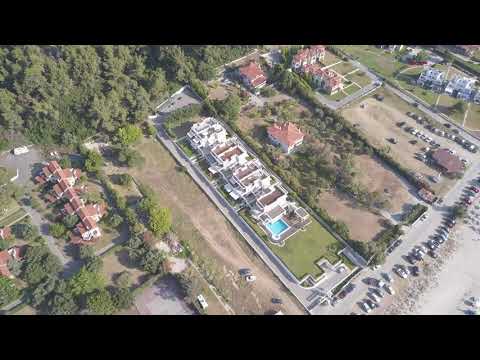This highly detailed aerial photograph, likely taken from a helicopter, airplane, or drone, showcases a sprawling, well-organized resort nestled in a picturesque valley surrounded by trees and hills. The resort features a number of white buildings with flat, tan or brown roofs, arranged in a series of gated sections. Notable structures include several three to four-story buildings, a large building surrounded by trees, and an even larger building with an ornate courtyard. A prominent feature near the front of the image is a blue, square swimming pool adjacent to one of the buildings, complemented by a jacuzzi in the bottom right corner. Roads and parking lots, filled with cars, wind through the resort, highlighting its accessibility. The image also captures a variety of residential-like structures, possibly duplexes or condos, which resemble small houses attached in a series. In the upper left corner, a hill covered in trees rises up, framing the lush, green landscape that encircles the resort.